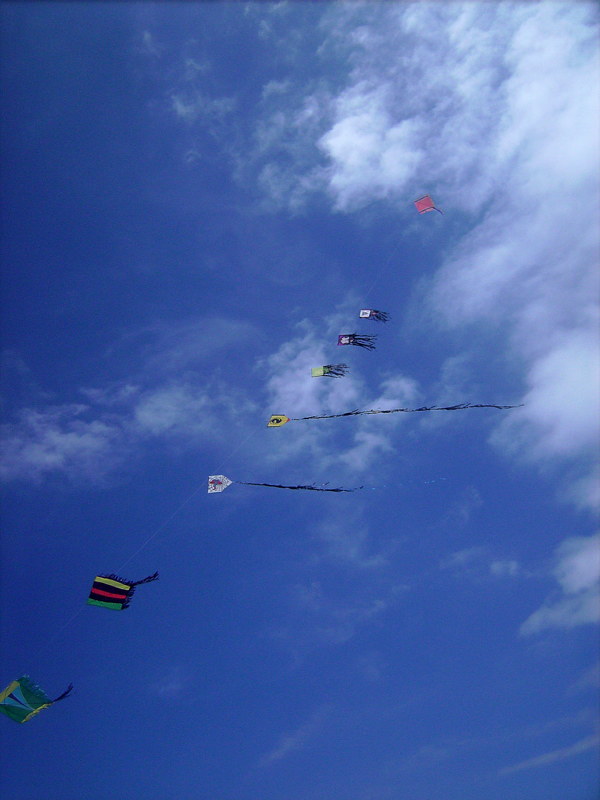In this image, a vibrant array of kites soars high against a bright blue sky mottled with white clouds. The kites are connected to a single string, flying in a diagonal line from the bottom left corner to the top right. The background features a gradient sky; the left side is a lighter blue with sparse cloud coverage, whereas the top right is marked by heavier clouds. Anchored at the bottom left, the first kite has green edges and a blue center with a purple streak. Next in line is a striped kite adorned with black, red, yellow, and green stripes. Further along, a white kite with a series of dots and a trailing black streamer fills the space. Following it, a yellow kite with black markings and an even longer streamer can be seen overhead. Higher up and to the right is a sequence of smaller, more distant kites: a yellow one with black streamers, a black one with black streamers, and another white one with black streamers. Among the assortment, a black and red striped box kite stands out with a short tail, and there is a pink kite at the farthest point in the sky. The collection showcases various designs, including box kites and traditional diamond shapes, united in a colorful display against the serene sky.